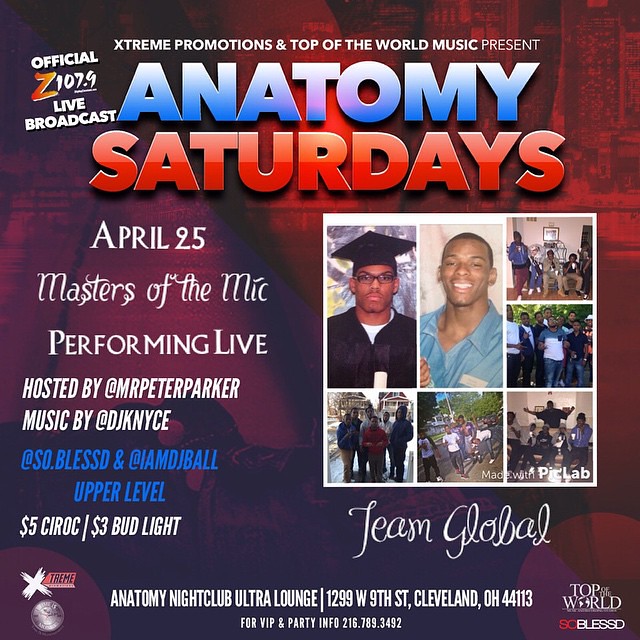This vibrant and energetic advertisement for a nightclub event "Anatomy Saturdays" features a red and blue color scheme with bold white text for clarity. At the top, it highlights the event sponsors with "Extreme Promotions and Top of the World Music Presents." The main headline, "Anatomy Saturdays," stands out prominently in blue and red font, announcing a special live performance by "Masters of the Mic" on April 25th, with an official live broadcast on 107.9.

The event is hosted by Mr. Peter Parker, with music provided by DJ K Nice, and will take place at So Blessed and Jamed Ball Upper Level. The advertisement includes specific details about the venue, "Anatomy Nightclub Ultra Lounge," located at 1299 West 9th Street, Cleveland, Ohio, 44113. It also mentions an enticing offer of $5 Seroke and $3 Bud Light to attract the crowd.

In the bottom right corner, additional sponsors "Top of the World" and "So Blessed" are listed. A collage of photographs featuring performers is positioned towards the bottom left, adding a personal touch to the advertisement. For more information on VIP and party arrangements, the contact number provided is 216-789-3442.

Overall, this advertisement effectively blends vibrant visuals and critical event details to capture attention and convey a festive nightclub atmosphere.